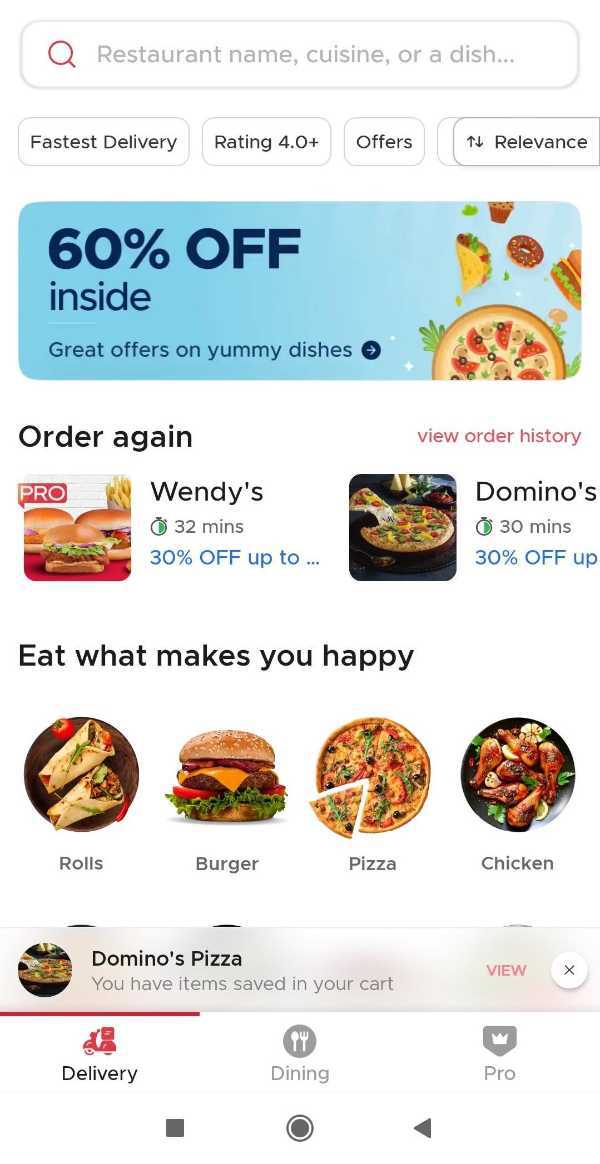The photo showcases a food-related app displayed on a cell phone in landscape orientation, set against a white background. The app interface is filled with various boxes, thumbnails, and icons. 

At the top, there's an oval or rectangular search box with rounded edges, featuring a gray border and white background. Inside the search box, a red magnifying glass icon is positioned on the left, followed by the gray text "Restaurant Name, Cuisine, or a Dish."

Beneath the search box are four selectable bubbles with gray or black text reading: "Fast Delivery," "Rating 4.0+," "Offers," and "Relevance."

A prominent light-blue banner with rounded edges and dark blue text displays, "60% Off in Sight, Great Offers on Yummy Dishes." Underneath this banner, a black heading reads, "Order Again," followed by thumbnails and descriptions for Wendy's (32 minutes) and Domino's (30 minutes, 30% Off Up).

Further down, a motivational message, "Eat What Makes You Happy," is flanked by circle thumbnail icons and text in black font for different food categories: "Rolls," "Burger," "Pizza," and "Chicken."

Towards the bottom of the interface, a gray transparent pop-up box appears, displaying: "Domino's Pizzas. You have items saved in your cart," along with a red "View" button on the right and a circle image on the left.

Finally, at the very bottom of the screen, there are navigation options for "Delivery," "Dining," and "Pro."